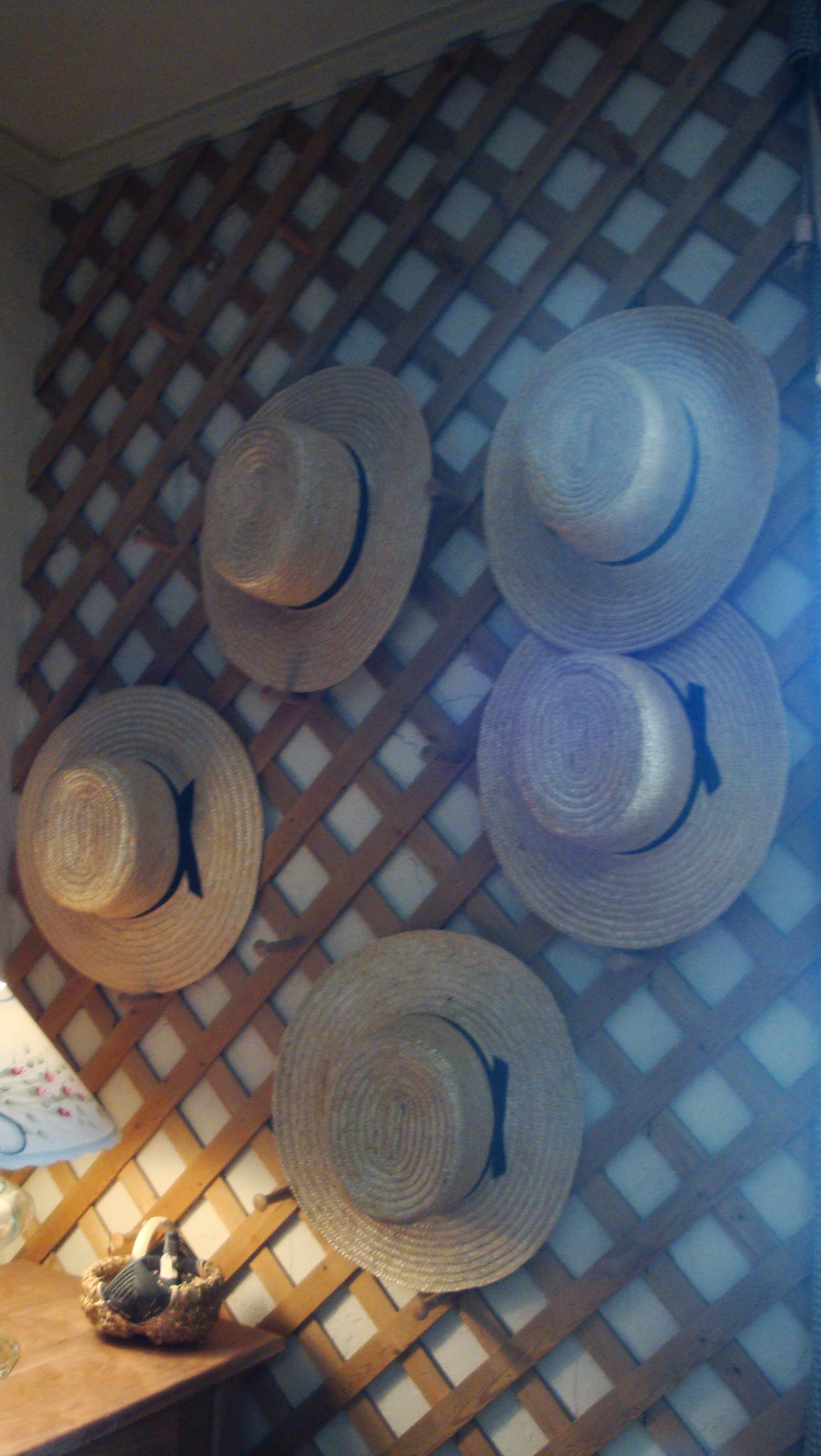This indoor photograph features a wooden lattice panel mounted on a white wall. Arranged in a circular pattern on the lattice are five light brown wicker sombrero hats, each adorned with a black ribbon around the base. To the lower left of the image stands a square wooden nightstand, upon which rests a lamp with a white shade featuring a flower design. Also on the nightstand is a yarn basket with a plastic handle, containing unidentifiable black objects. The lamp provides the primary illumination for the scene, casting a soft light over the rustic and decorative arrangement.